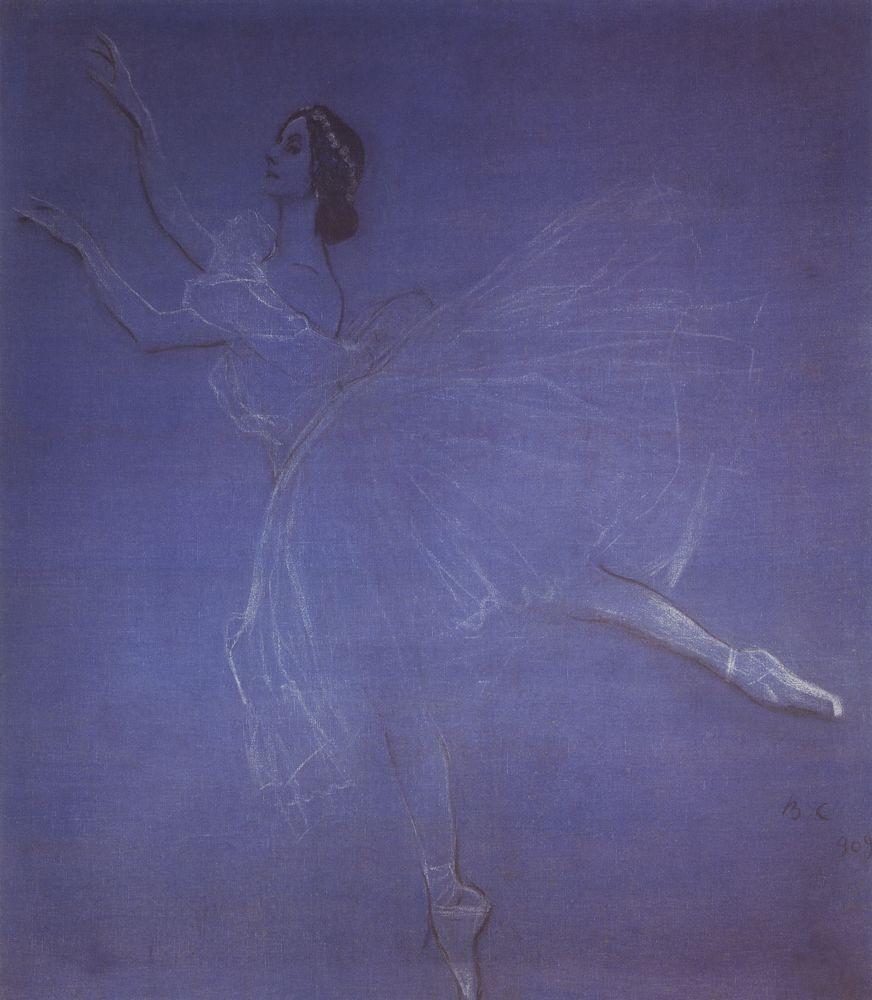This image depicts a delicate and ethereal sketch of a ballerina captured in mid-performance. Set against a muted, deep blue-gray background, the ballerina's form is defined through faint yet expressive outlines that convey both depth and movement. She stands gracefully on one toe, her other leg extended behind at a pronounced angle, accentuating her poised balance. Her arms reach out elegantly toward the upper left, accentuating the flow and daintiness of her motion.

Her attire, a lightly drawn tutu and frilly ballet dress, is rendered in soft shades of white and light pink, further highlighting the delicate nature of the sketch. The neckline of her dress is notably low-cut, with frill details adding to her refined appearance. Her dark hair is styled into a bun adorned with a row of flowers or possibly a crown of jewels, extending from her forehead down to the nape of her neck, giving her a regal yet delicate elegance. The subtleties in the ballerina's form, from her slightly arched back to the faint yet noticeable earrings, contribute to the overall softness and daintiness of this youthful dancer.

The use of predominantly black and white marks contrasts gently with the deep background, enhancing the transparency and ethereal quality of her outline, making her appear almost as a whisper of a figure against the vast muted canvas.